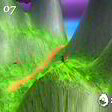The image is a small, square-shaped snippet of gameplay, showcasing a mountainous terrain with gray, mountain-like structures adorned with patches of green grass. The top of the image features a "07" in white font. The landscape is further accentuated by strips of red, yellow, and orange hues, adding to the scenic diversity. The sky above transitions into a blend of purple and blue tones, creating a striking backdrop. A small white icon is visible in the foreground, accompanied by a white glare effect that permeates the entire image. The green shades vary between lighter and darker tones, enhancing the depth and texture of the environment.